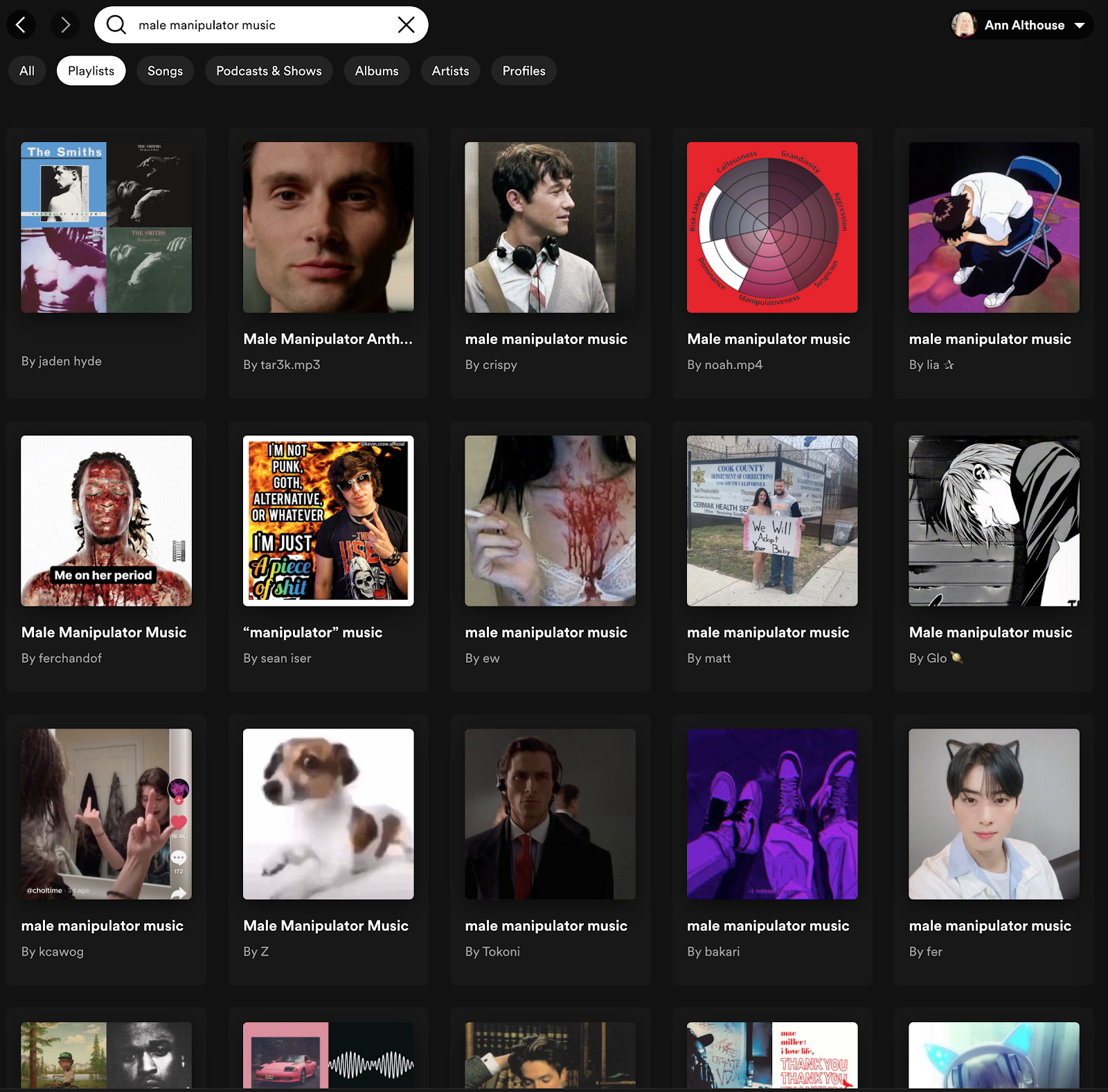The screenshot features a music streaming interface. In the search bar, "male manipulator music" is typed. To the right, there is a section labeled "In Our Art House," showing an album cover with a woman's picture. At the top of the interface, various tabs such as "All," "Playlists," "Songs," "Podcasts and Shows," "Albums," "Artists," and "Profiles" are displayed, with the "Playlists" tab being highlighted with a white, rounded rectangle. The word "Playlists" is in black text, standing out against the white background. Below this, several playlist thumbnails are visible, each titled "male manipulator music," with one variant listed as "male manipulator 'music'" with "manipulator" in quotation marks. The titles of additional songs or playlists are partially cut off at the bottom of the screenshot and are not fully readable.